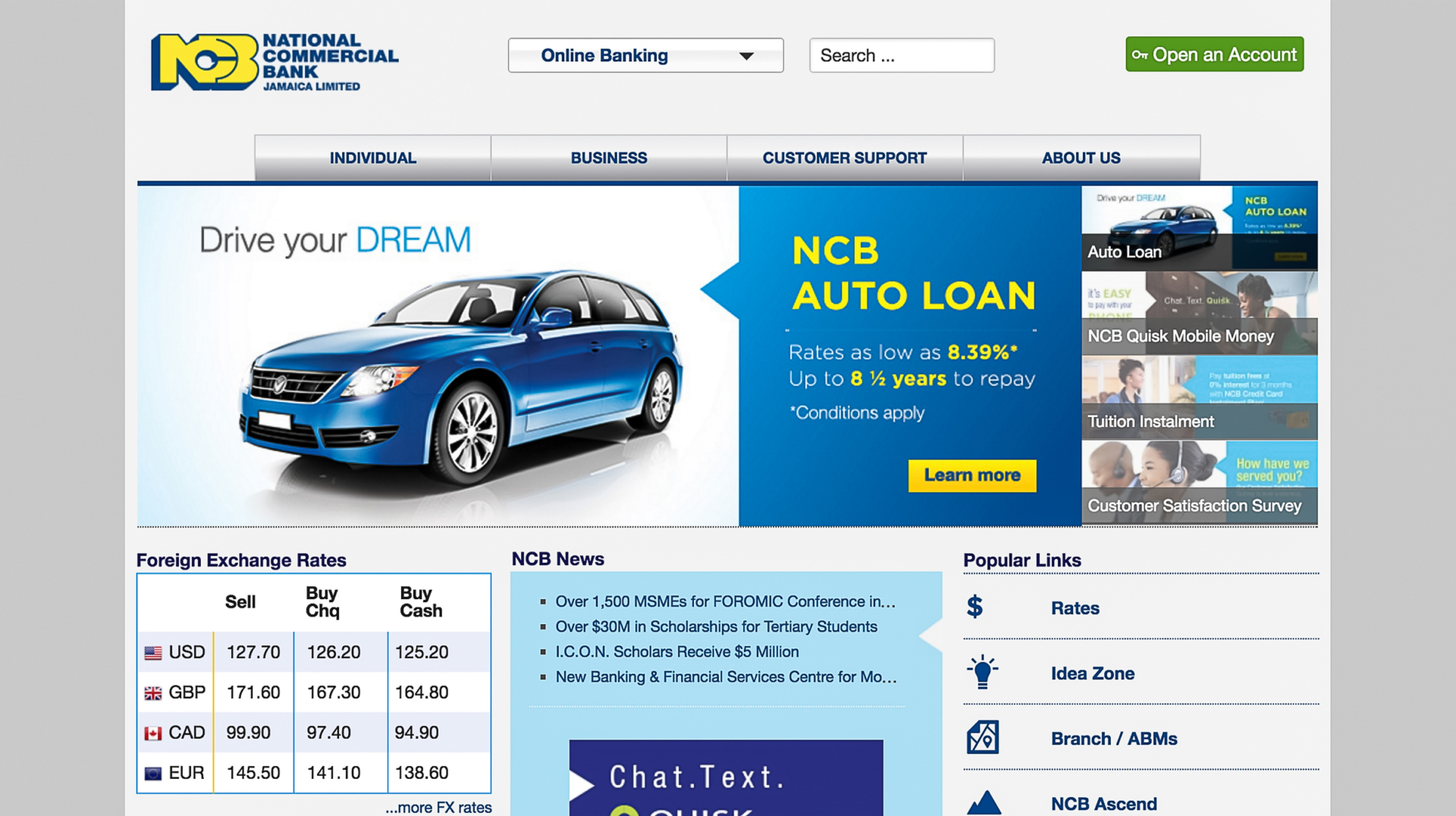The image has a gray background and prominently features the logo "NCB" in yellow, alongside the full name "National Commercial Bank, Jamaica Limited" in blue. Below the logo, there are interactive elements including an online banking search option and an "Open an Account" button, which is displayed in white text on a green rectangle.

At the top of the image, there are four navigational tabs in gray, each labeled in blue text: "Individual," "Business," "Customer Support," and "About Us." Below the tabs, a promotional section showcases a tagline "Drive Your Dream" with the word "Dream" highlighted in blue, accompanied by an image of a blue car.

The promotion highlights NCB's auto loan offer, with the loan rate displayed as "NCB auto loan rate as low as 8.39%" in yellow text. Additional details include a repayment period "up to 8 1⁄2 years" also in yellow, and a fine print note marked by an asterisk stating "conditions apply." There is a "Learn More" button in blue text on a yellow rectangle.

To the right of this promotion, there are four distinct sections with headings: "Auto Loan," "NCB Quisk Mobile Money," "Tuition Installment," and "Customer Satisfaction Survey." Additionally, there is a list of popular links, including "Rates," "Idea Zone," "Branch/ABMs," and "NCB Ascend."